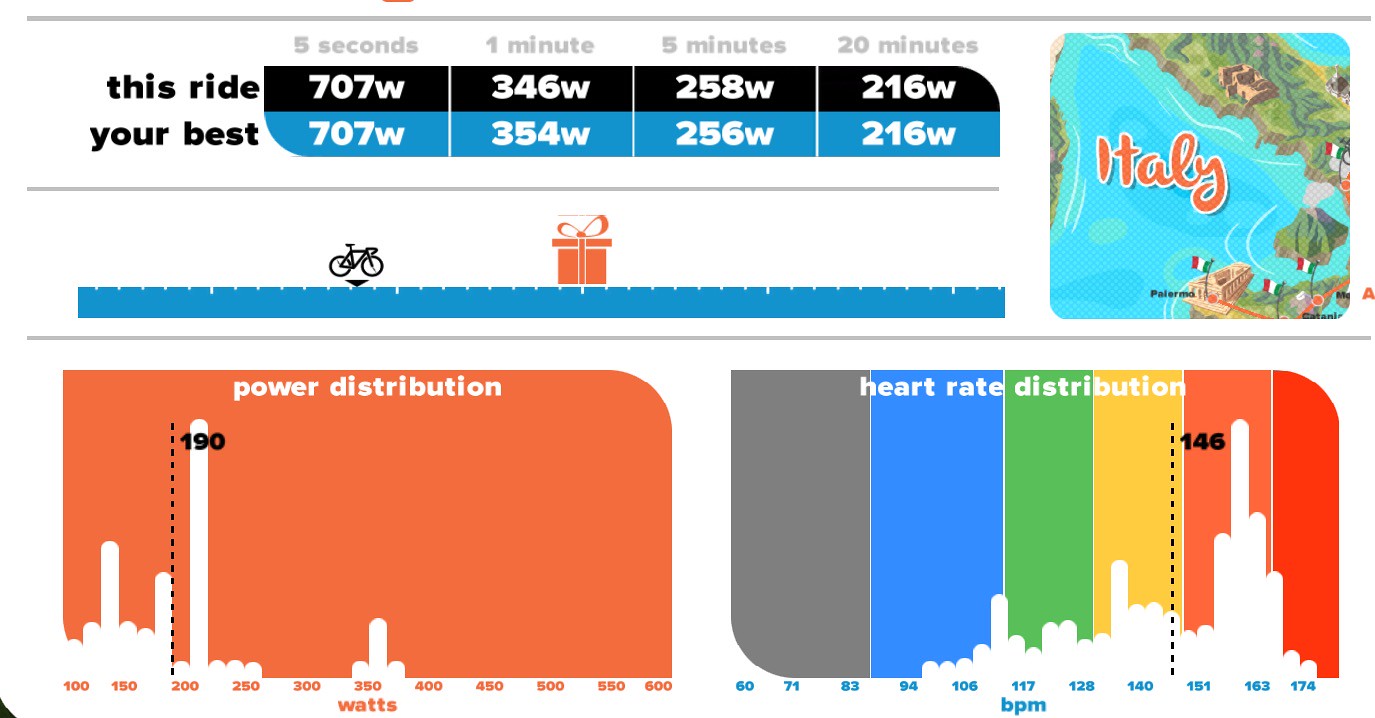The image is a detailed screenshot from a cycling workout app, displaying various performance metrics and geographic information. At the top, the chart is divided into different time intervals: 5 seconds, 1 minute, 5 minutes, and 20 minutes. Below these intervals are wattage readings for "This Ride" and "Your Best": 707W, 346W, 258W, and 216W for "This Ride," and 707W, 354W, 256W, and 216W for "Your Best." In the lower section, there's a small illustration of a bicycle moving toward an orange present icon, accompanied by a ruler-like graphic. To the right of this, in the upper corner, is a label with "Italy," featuring a map, a flag, a body of water, mountains, and houses.

Further below, the app provides two distinct graphs. The first graph, titled "Power Distribution," has an orange background with white bars and measures power output in watts. The second graph, labeled "Heart Distribution," displays heart rate data in a color gradient ranging from green and blue to yellow and red, mapping beats per minute. The overall aesthetic of the app includes a mix of cartoonish fonts and detailed analytics, merging both fun and informative elements.